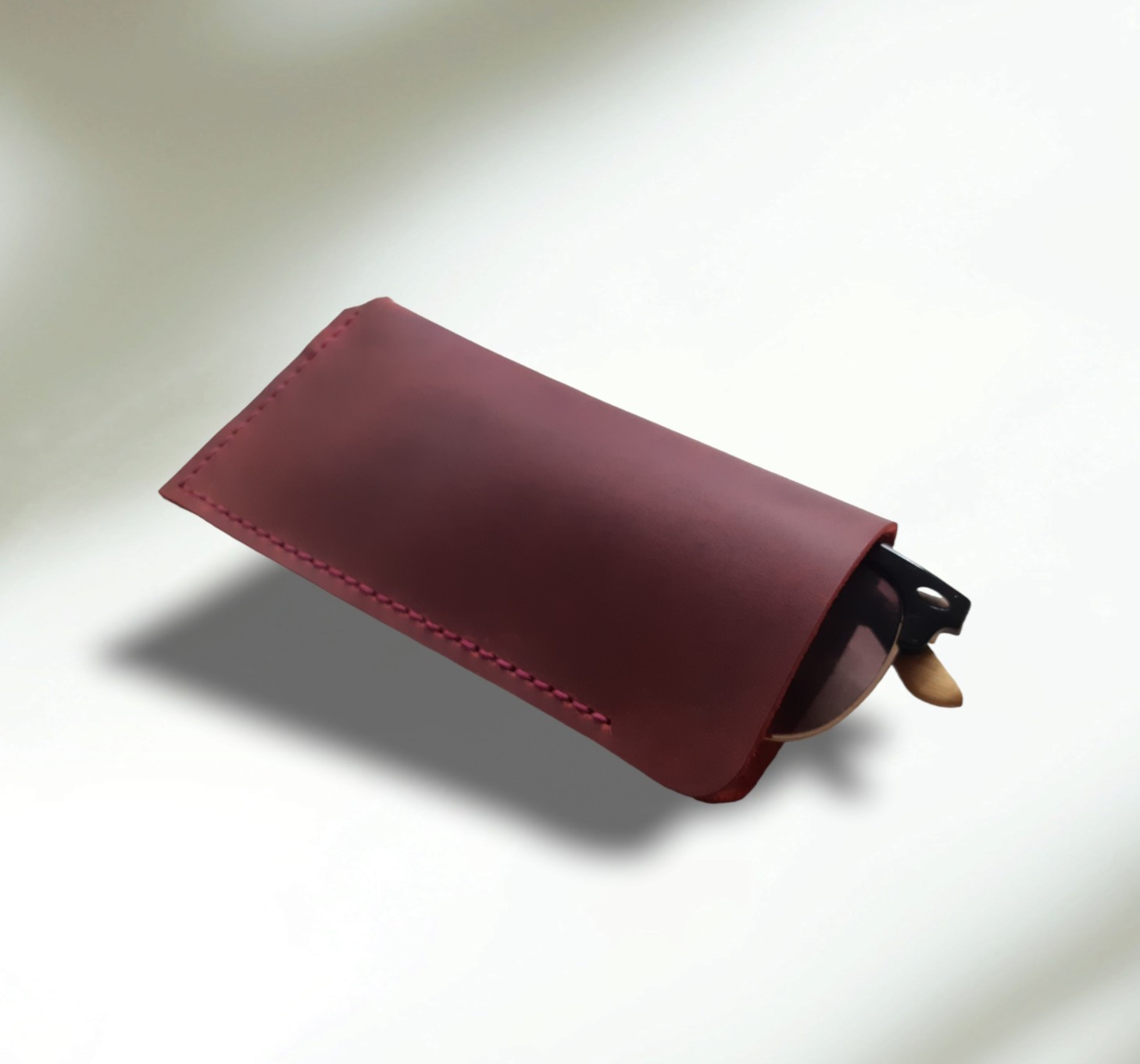The image is a professionally staged, full-color photograph taken indoors using artificial light, set against a predominantly white background that includes some shaded areas in the lower right and upper left. Dominating the scene is a pair of lightly tinted sunglasses with a black and brown frame. The glasses are partially placed inside an eyeglass pouch, revealing just a hint of the frame and a third of the lenses. The pouch itself is crafted from a rich crimson, burgundy, or raspberry-colored material, accentuated with reddish stitches along the bottom. There's a shadow of the case visible on the white surface, highlighting the sophisticated and likely expensive nature of the sunglasses and their carrier.